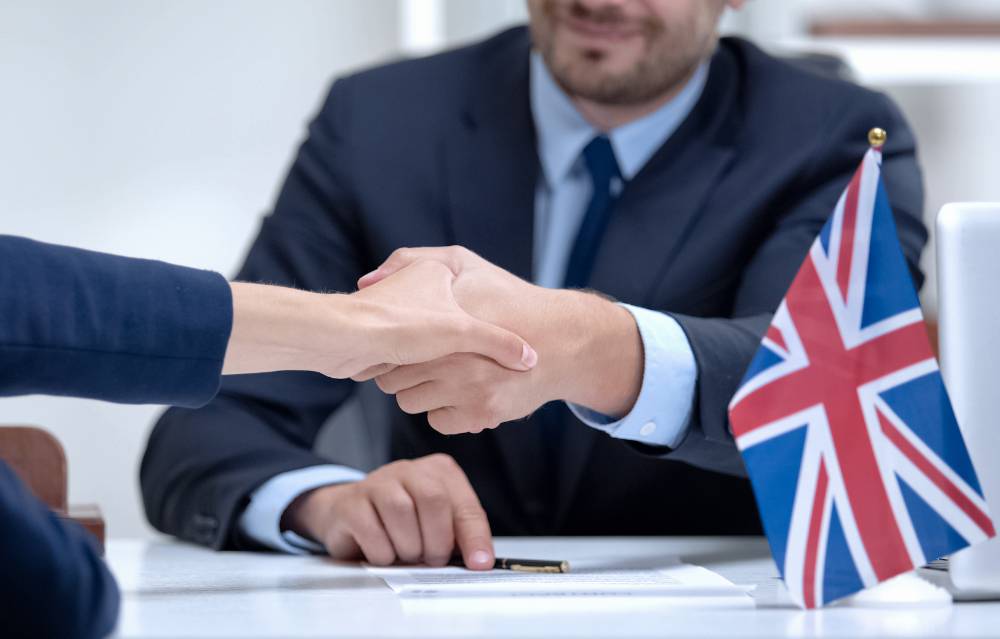In this photograph, a man dressed in a navy blue suit, a light powder blue dress shirt, and a dark blue tie is shaking hands with a woman. The handshake occurs with his left hand, while his right hand rests on a white desk, holding a pen over a piece of paper that appears to have writing on it. The man, who is smiling, sports a short beard and mustache. A small British flag is prominently displayed in the foreground on the right side of the desk. The woman’s appearance is limited to her left hand, identifiable by her fingernails, as the rest of her is cropped from the image. The scene is set in a white room with a white desk and a white shelving unit behind the man.